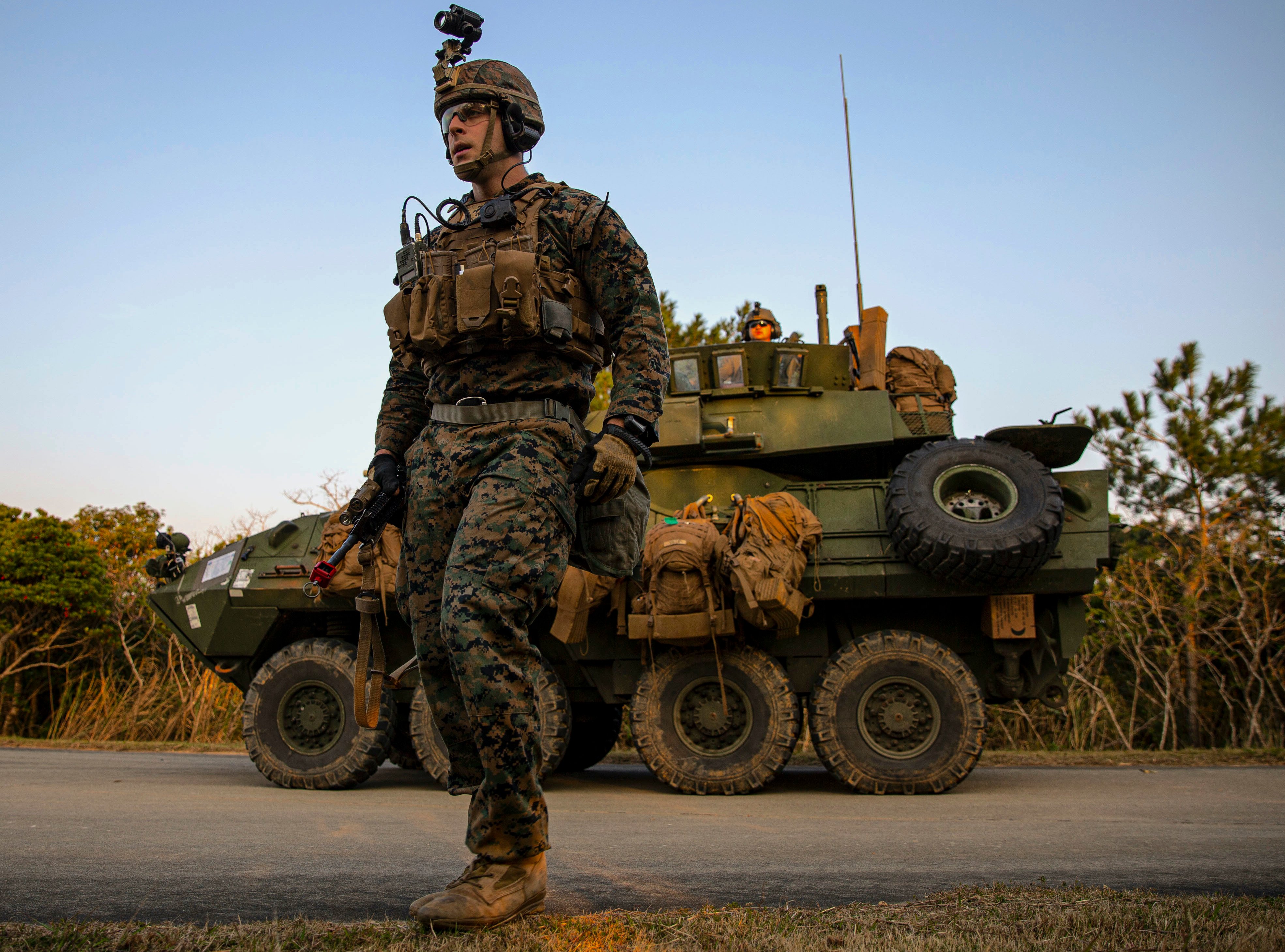In the photograph, a soldier in camo fatigues walks to the left side of the frame. He wears a helmet with a chin strap and an attached video camera, as well as glasses. Over his chest, he has a utility vest with numerous pockets, one of which appears to hold a walkie talkie. The scene features a green, armored vehicle with eight wheels (four on each side) in the background, vaguely resembling a Humvee. A spare tire is visible on the vehicle's side, and another individual is seen emerging from it. The backdrop includes sparse vegetation, such as some grasses and a few trees, set in what appears to be a mostly barren area. The overarching colors in the image include green, beige, dusty brown, black, and touches of blue and orange.